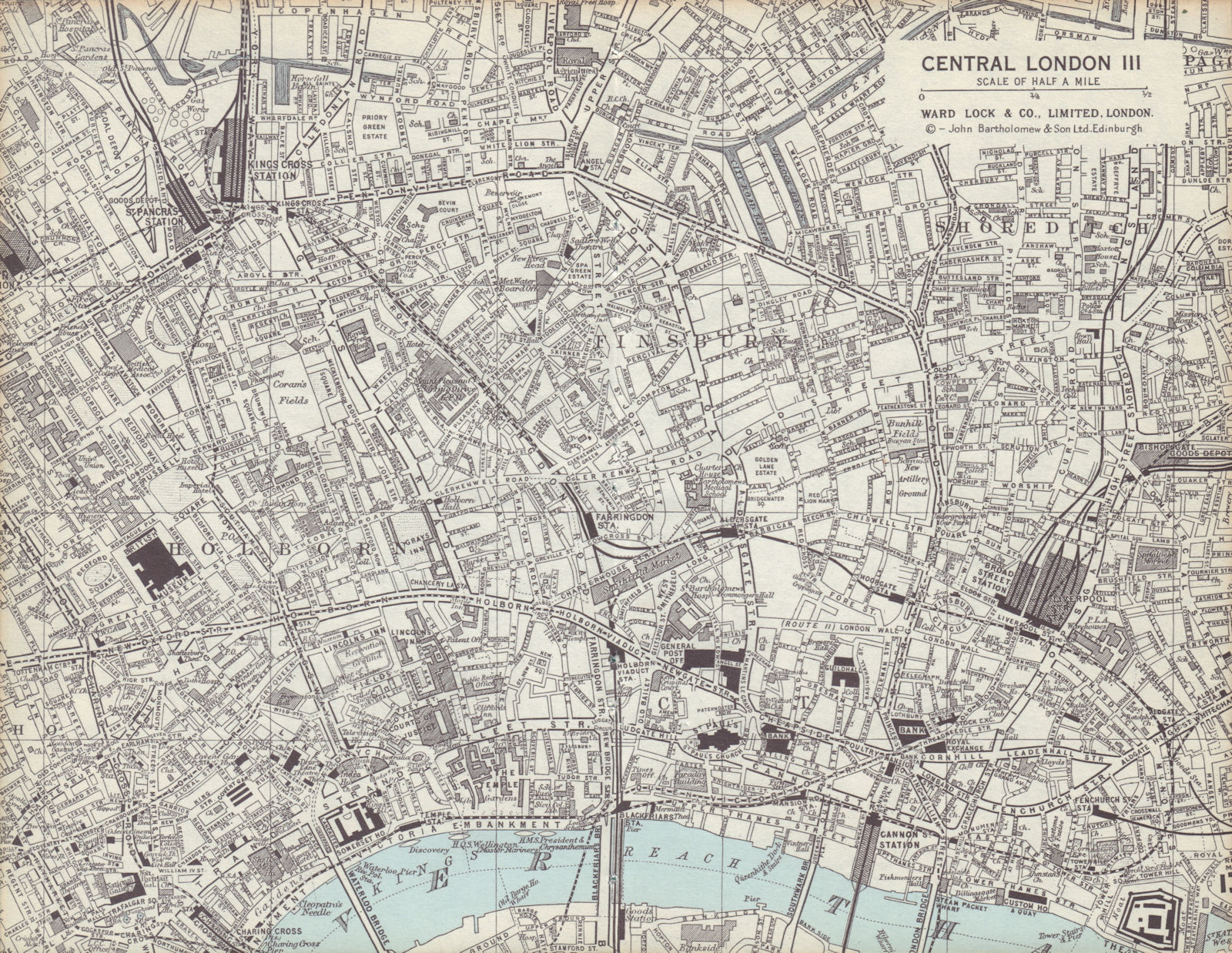This is a historic, detailed map of Central London that prominently features key locations such as Finsbury, Shoreditch, Holborn, Broad Street Station, King's Cross Station, and the British Museum. The map is copyrighted and produced by Wardlock & Co. Ltd. London, with cartography by John Bartholomew & Son Ltd. Edinburgh. In the upper right corner, the map is labeled "Central London III" with a scale of half a mile. The River Thames, depicted in a light blue color, cuts across the bottom center of the map, with several bridges spanning the water. The majority of the map is rendered in black and white, with certain areas shaded in darker grey tones, indicating the dense urban layout.